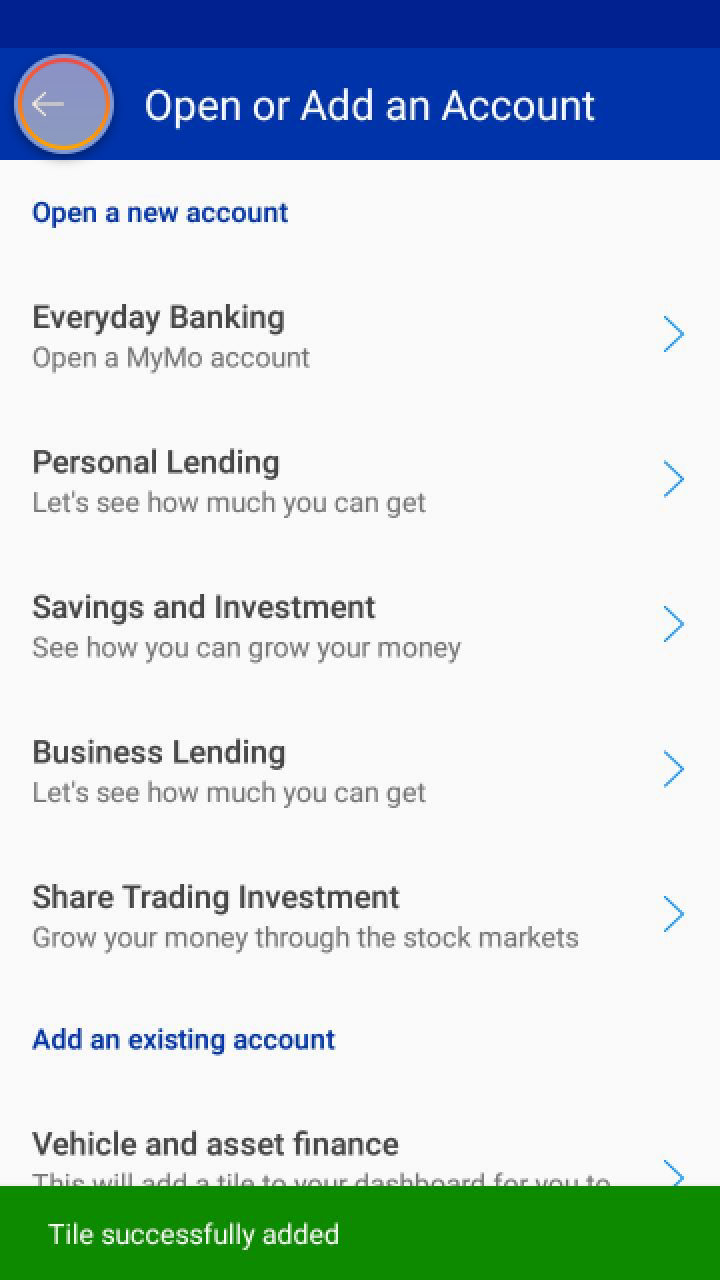The image is a screenshot from a website featuring a structured design with various sections and color elements. At the top, there's a dark blue banner that transitions into a slightly lighter blue background just below it. A prominent gray circle occupies the center area, containing a left-pointing white arrow. Within this gray circle, there are two segments in different shades of orange—one darker and one lighter.

In white text, the phrase "Open or Add an Account" is displayed prominently, with the 'O' in "Open," 'A' in "Add," and 'A' in "Account" capitalized. Below this, a button-like section with a gray background and blue text reads "Open a New Account," with the 'O' capitalized.

As the content flows downward, various service options are listed, each accompanied by a right-pointing arrow. The options are:

1. Everyday Banking - "Open a MIMO Account" (with 'MIMO' stylized as "MYMO").
2. Personal Lending - "Let’s see how much you can get."
3. Savings and Investments - "See how you can grow your money."
4. Business Lending - "Let’s see how much you can get."
5. Share Trading Investment - "Grow your money through the stock markets."

Another button with blue text on a gray background is present, stating "Add an Existing Account," where the 'A' is capitalized. 

Further down, in black print, the section "Vehicle and Asset Finance" is visible. However, some of the text in this section is obscured by a green banner with white text that reads "Tile Successfully Added."